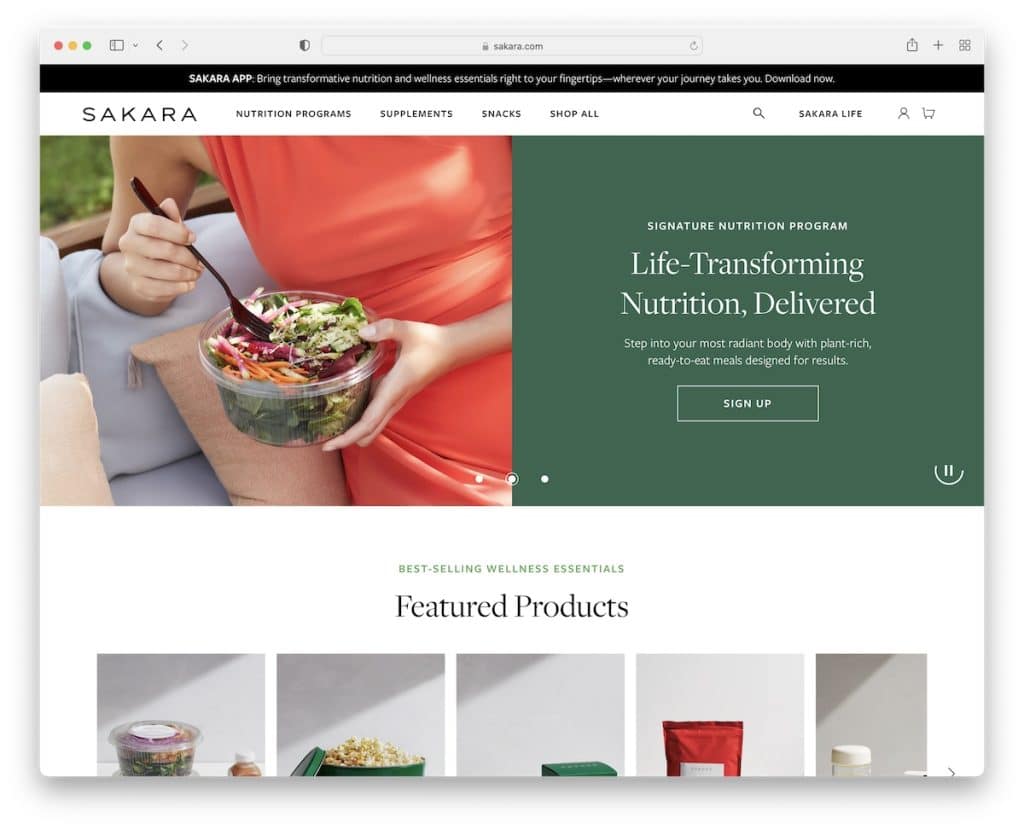This is an image of the homepage of the website "SAKARA," a platform dedicated to promoting a healthy lifestyle. The header of the site prominently features a call to action: "Sarah App, bring transformative nutrition and wellness essentials right to your fingers wherever your journey takes you. Download now." A white navigation bar immediately below offers links to various sections: "Sakara Nutrition Program," "Supplements," "Snacks," and "Shop All," under the overarching category, "Sakara Life." Icons for search, user profile, and shopping cart are located on the right side of the bar.

Just beneath this navigation, there is a central image of a woman in a red top that extends below her waist, possibly a dress. She is enjoying a salad from a Tupperware container while seated on a gray couch adorned with throw pillows. The setting includes a wooden element and a visible grassy background, creating a serene atmosphere. 

To the right of this image, bold text reads, "Life Transforming Nutrition Delivered, Signature Nutrition Program. Step into your most radiant body with plant-rich, ready-to-eat meals designed for results." A conspicuous green button labeled "Sign Up Now" invites visitors to enroll in the nutrition program.

At the bottom section of the image, the text "Best Selling Wellness Essentials, Featured Products" introduces a showcase of various items. Among the featured products are snacks such as popcorn and yogurt, though some items, like a red bag and a bottle with a white top, are partially cut off, indicating a larger collection of wellness products available for purchase.